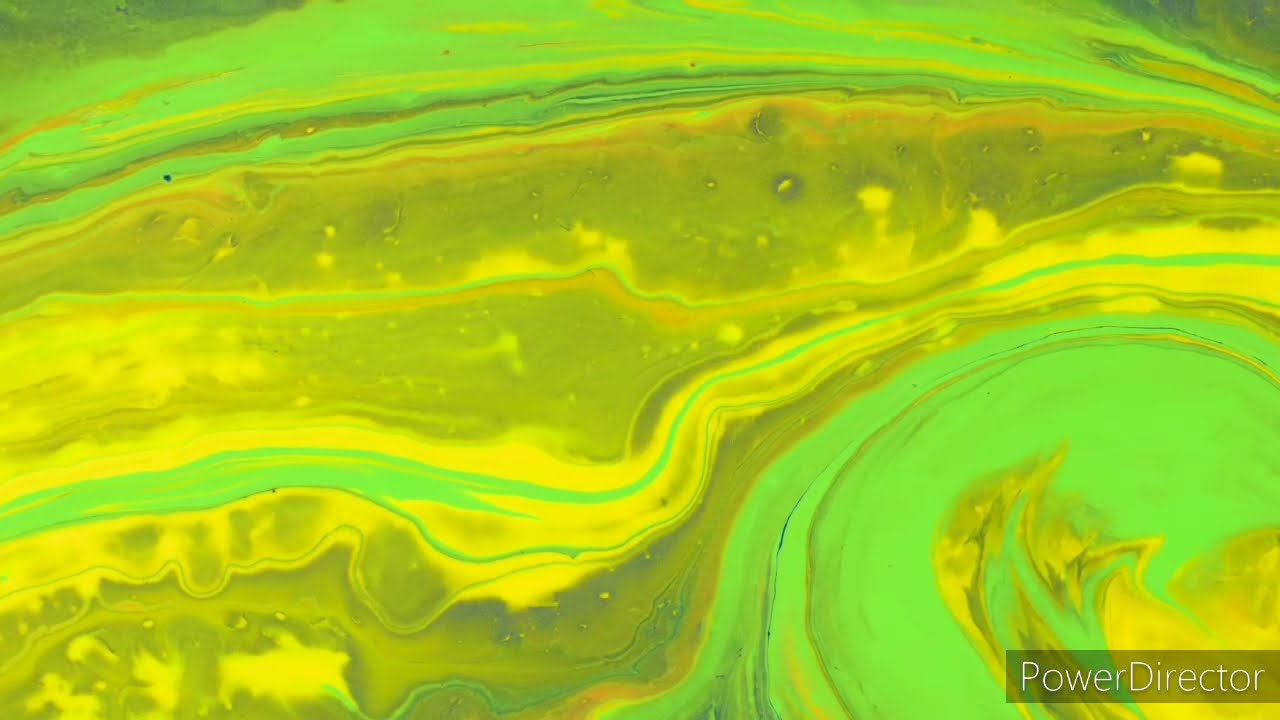The image features intricate swirls and patterns predominantly in shades of green and yellow, with touches of orange and gray. The colors blend and twist in a manner reminiscent of liquid flow, such as poured paint swirling together or a type of imaging. Bright neon green and lime green are prominent, interspersed with areas of bright yellow and softer, almost drifting yellow. The swirls create ornate patterns, bending and curling into streams and patches that appear darker and lighter, suggesting a dynamic flow. Notably, in the bottom right corner, there's a white font text that reads "Power Director," indicative of the software used for editing.